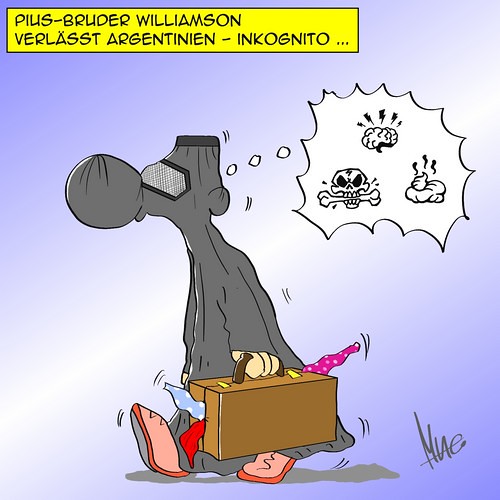This cartoon features a yellow rectangle at the top with a black border, bearing the text "Pius Bruder Williamson for last Argentinian incognito." Beneath this header is a white starburst, also outlined in black, containing icons that represent various thoughts. These icons include a brain, a skull and crossbones, and what appears to be a small pile of poop. These thoughts are enclosed within a jagged-edged thought bubble. The pondering creature depicted below has an exaggeratedly large nose and is adorned in a dark gray cape. It is walking leftward across the frame, seemingly moving away from the image's right side.